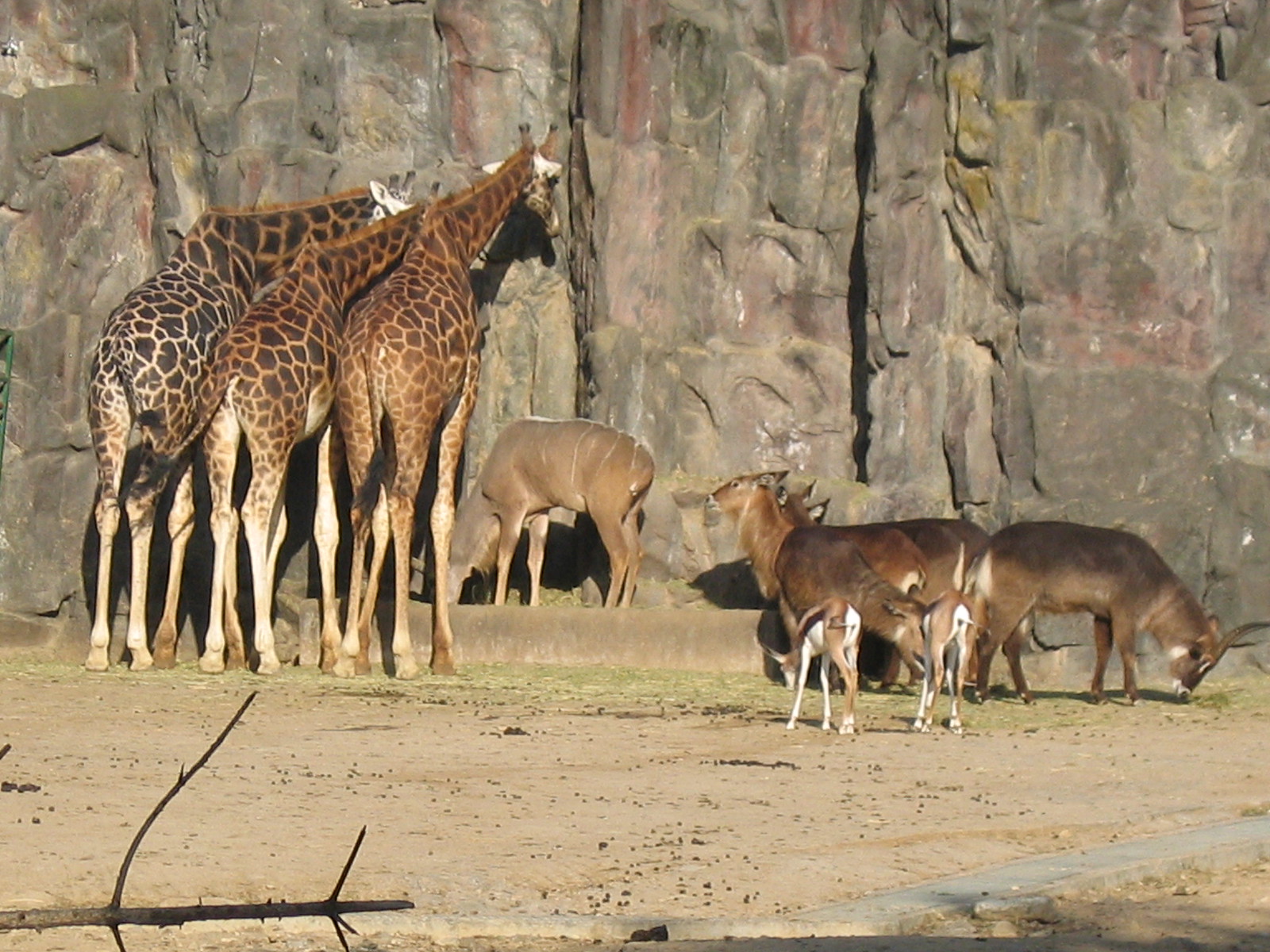In the color photograph, a group of animals is gathered in a sandy, dirt field with sparse tufts of grass. Prominently on the left, three majestic giraffes stand closely together, their sides touching and tails pointed towards the camera as they face a rugged, grey rock wall streaked with patches of red, yellowish-green, and white. The giraffe on the far left is darker, almost black, while the other two exhibit a lighter honey-brown hue. All giraffes have distinctive patterned coats, long legs, and short manes, and the characteristic ossicones on their heads.

To the right of the giraffes, a group of smaller quadrupeds, possibly goats or gazelles, includes at least four adults and two young ones. These animals, varying in shades of light to darker tan, are dispersed and engaged in different activities like grazing and looking at the giraffes. Notably, one of the smaller animals stands on a small ledge just behind the giraffes, adding depth to the scene.

The ground is predominantly sandy with minimal grass, and in the foreground, a large tree branch lies on the lower left, while a shallow trough or puddle of water is visible on the lower right. The combined presence of these animals and the rocky background creates a harmonious and serene wildlife exhibit scene.